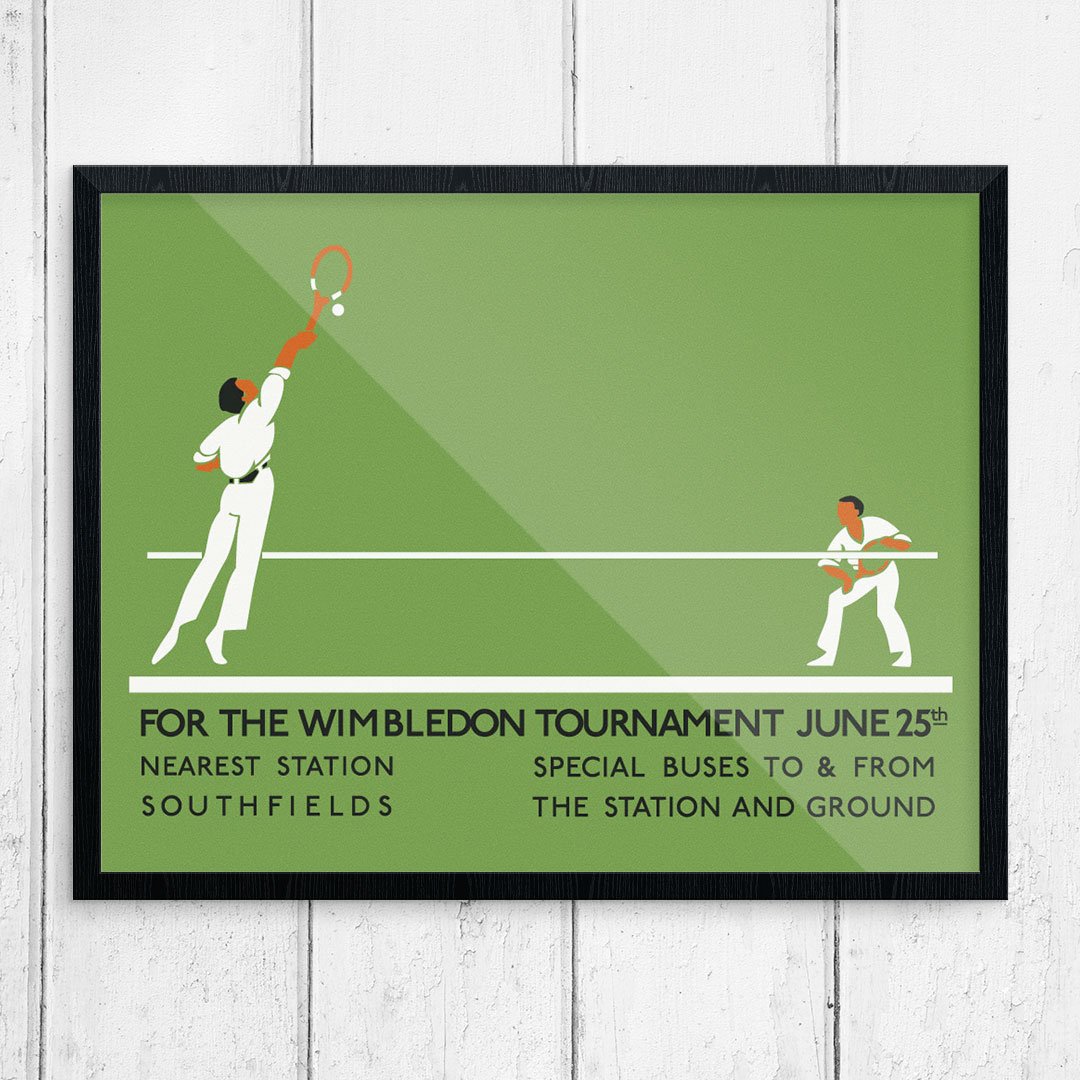This detailed image depicts a framed artwork with a black border. Inside the frame, the background is split diagonally into two green horizontal triangles, with the left triangle being slightly darker than the right. Central to the image are two white horizontal lines, which suggest the net on a tennis court. On the left side, a person dressed in all white is shown leaping to hit a tennis ball with a racket, while on the right side, another person in white stands poised, also holding a racket. Beneath the lower white line, black text announces “For the Wimbledon tournament June 25th, nearest station Southfields, special buses to and from the station and ground.” The framed artwork, likely a promotional piece for the Wimbledon tournament, is set against a white wood-paneled backdrop.